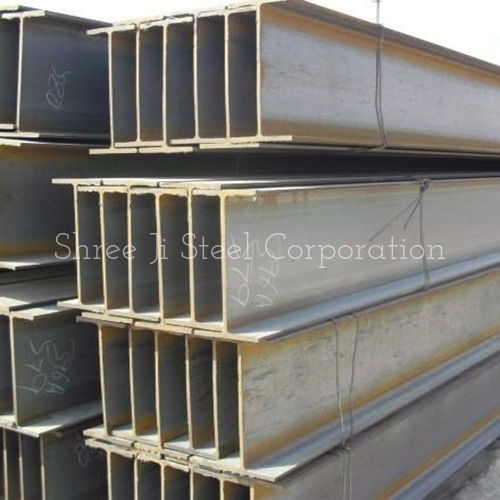This photograph captures a construction site where numerous silver steel I-beams are meticulously stacked atop one another. The central focus of the image is the prominently displayed white text that reads "Shri G. Steel Corporation." Each I-beam is visibly weathered, showing signs of rust and various scrapings, indicating their rough use over time. Along the beams, numbers such as "396A579" can be seen, suggesting a system of identification. The beams are arranged in stacks four high and six wide, creating a structured and organized pile. Their perpendicular placement allows for a clear view halfway down the length of the beams, showcasing their size and the meticulousness of their arrangement. Shadows and shading within the image add depth, emphasizing the industrial atmosphere of the construction site.